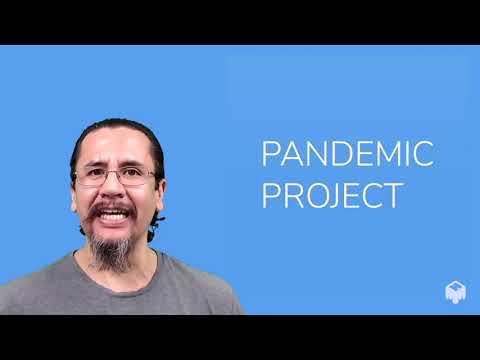The image appears to be a still from a presentation video, featuring a pale blue background framed by black bars at the top and bottom. On the left side, there's an older man with a caramel-colored complexion and long, black hair pulled into a ponytail. His facial hair includes a thin black mustache and a salt-and-pepper beard, extending from his chin. He wears thin metal-framed glasses and a gray crew neck shirt. The man is captured mid-sentence, with his mouth slightly open, as if speaking to the camera. The lighting, likely from above, adds a slight shine to his forehead and cheeks. On the right side of the image, in all-caps white sans-serif font, the text reads "PANDEMIC PROJECT." Additionally, in the bottom right corner, there is a white logo depicting a stylized cartoon toaster.